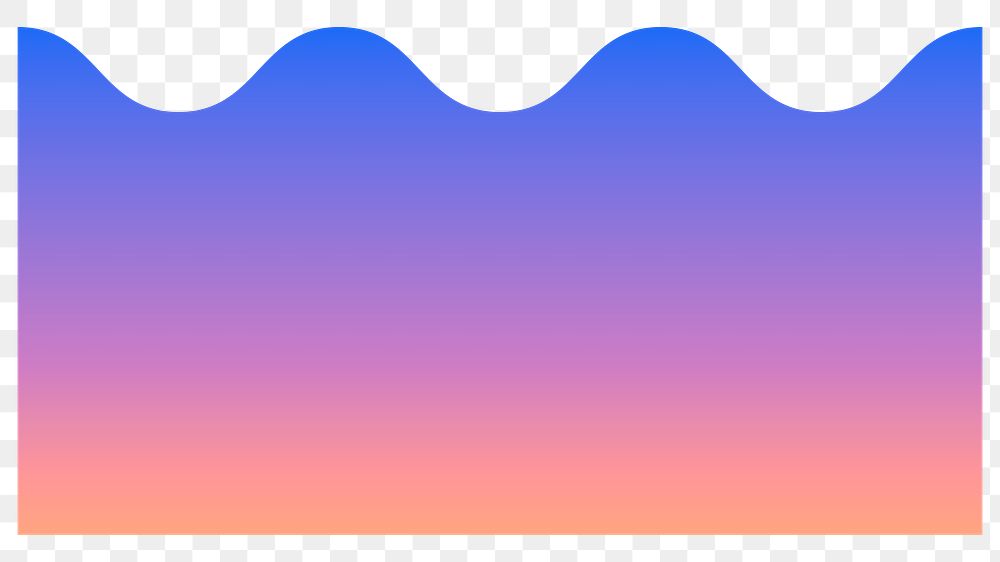This image features a low-quality graphic with a digitally-created design, commonly used in web or graphic design projects. The background consists of a gray and white checkerboard pattern, a common indicator for transparency in image editing. Centered in the middle of this transparent background is a wavy design pattern that transitions in color from top to bottom. The wave pattern starts with blue at the top, shifts to a purple that leans more towards red in the middle, and finally transitions into a pinkish-orange-red hue at the bottom. The waves are characterized by their peaks and valleys—specifically, there are two full peaks and two half peaks with three valleys. The overall style of the image is calm and neutral, suitable for backgrounds or foundational elements in design work. The image contains no text or other objects, purely serving as a design element to be further manipulated or integrated into a larger project.